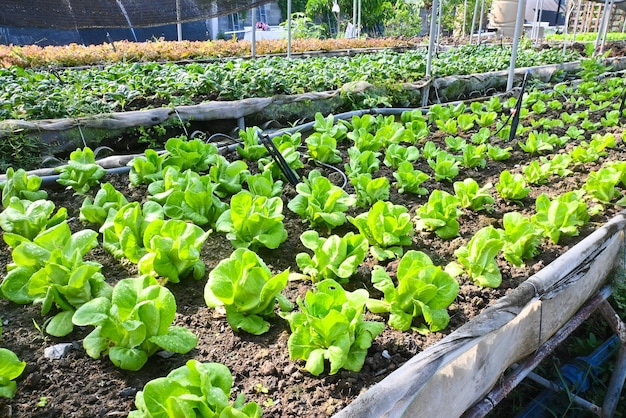The image depicts an orderly and well-maintained garden or farming area, visually resembling a greenhouse setup. At the forefront are several long, elevated beds or steel boxes filled with various types of leafy greens and young plants. The central bed is prominently filled with large, pale green leaves, likely butter lettuce or bib lettuce, growing in nutrient-rich soil. These beds are framed with materials such as burlap and supported by stakes, indicating a structured cultivation method. There are two or three rows of these beds stretching into the background, where the greenery appears darker, suggesting different types of plants like spinach. In the very back, there is a section with yellowish vegetation, possibly wheat or a different type of grass. The overall impression is of an organized agricultural space dedicated to starter plants, likely in the early stages of growth, awaiting transplantation to more spacious grounds for full development.